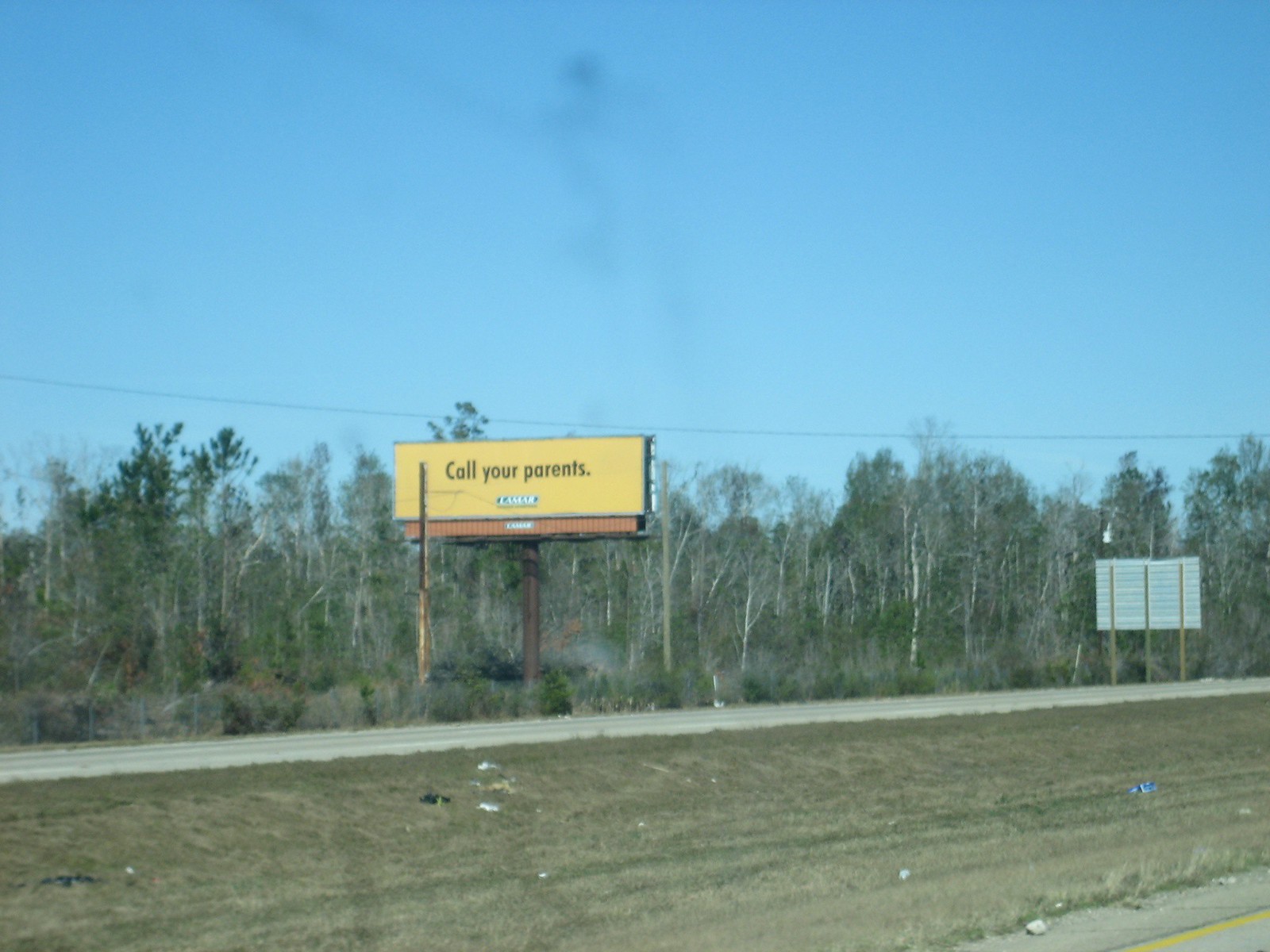The photograph captures a sprawling countryside scene viewed from the side of a rural road. Dominating the image is a large, mustard yellow billboard mounted on either wooden or metal posts, standing prominently against a backdrop of dense trees. The billboard displays a stark black message that reads "CALL YOUR PARENTS" in bold lettering, with additional, smaller text in a blue box below that is illegible. At the forefront, the road is visible with a yellow center stripe, suggesting a divided highway with traffic flowing in the opposite direction. A grassy median separates the two lanes, and scattered litter can be seen among the vegetation, including blue, white, and black debris. The sky above is clear and blue, unbroken by clouds except for a small, indistinct black mark, possibly smoke. To the right of the billboard is an additional road sign facing away from the camera, adding to the sense of depth in this expansive, tranquil, yet somewhat desolate rural landscape. The trees in the background are mostly barren, implying a fall or winter setting. Telephone lines are visible stretching across the blue sky.